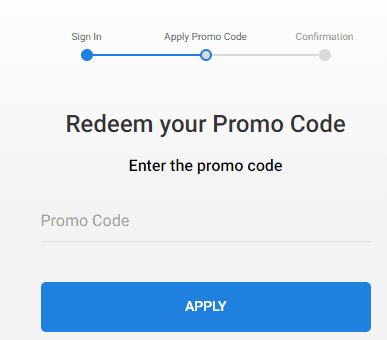The image features a light blue background with a central interface for applying a promo code. The interface displays a progress tracker consisting of a sequence of blue and gray elements indicating different stages. The top section is a very light blue box with the text "Sign In," followed by "Apply Promo Code" and "Confirmation." 

A solid blue dot marks the "Sign In" stage, connected by a deep blue line to a blue-outlined dot representing the "Apply Promo Code" stage. This line then turns gray, leading to a gray dot which indicates the "Confirmation" stage. 

Below this, the interface prompts users with the instruction "Redeem Your Promo Code." Beneath this instruction is a text field labeled "Enter the Promo Code," framed by a horizontal line where users can input their code. At the bottom of the interface is a substantial blue button labeled "Apply" in white text. This visually guided process emphasizes that the user has successfully signed in but still needs to enter and apply their promo code before reaching the confirmation stage.